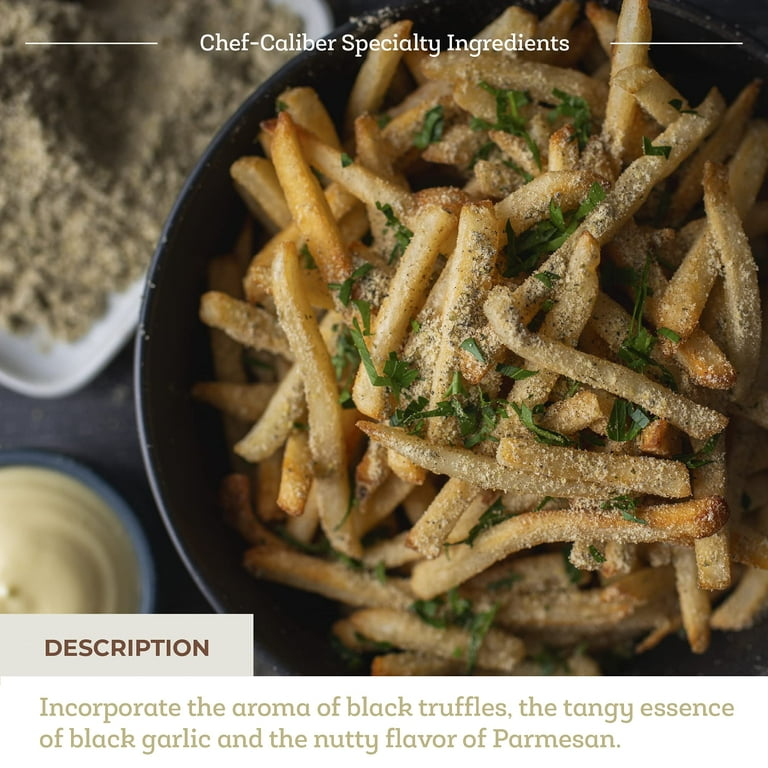This close-up photo showcases a mouth-watering bowl of shoestring-cut garlic fries, nestled inside a black pan. At the top of the image, "Chef Caliber Specialty Ingredients" is prominently displayed. The fries are adorned with assorted ingredients, including a powdery layer of Parmesan, the earthy aroma of black truffles, tangy black garlic, and garnished with green sprigs of cilantro. The fries appear lightly fried, almost as if freshly cut and quickly pan-seared. In the background, the image subtly hints at other accompanying dishes, such as a muted plate of what could be brown rice and a small black dish containing a yellow substance that resembles butter. Below the main image, a description box emphasizes the rich flavors incorporated into the dish: "the aroma of black truffles, the tangy essence of black garlic, and the nutty flavor of Parmesan."